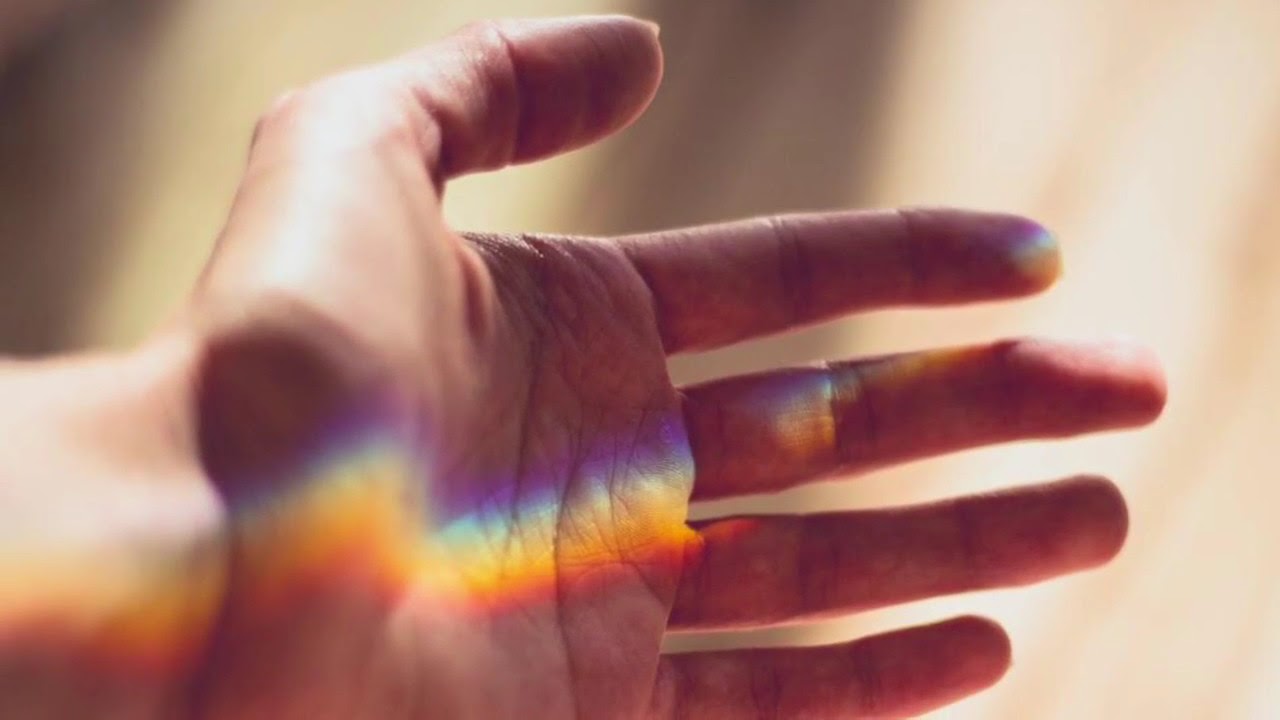The image is a close-up photograph of a light-skinned, outstretched left hand, prominently displaying long fingers and a portion of the thumb with visible creases and fine wrinkles. The focal point of the image is the vibrant rainbow-colored light reflecting on the hand, stretching from the top to the bottom of the palm. The rainbow's colors transition smoothly from purple at the top, through blue, green, yellow, and orange, to red at the bottom. The background is a blurry, bright tan or cream color, suggesting direct sunlight and daytime conditions. Subtle shadows and the brightness of the surroundings enhance the vividness of the rainbow effect on the palm. Only a small portion of the wrist is visible in the lower left corner, emphasizing that the main focus is on the hand and the colorful light play upon it.